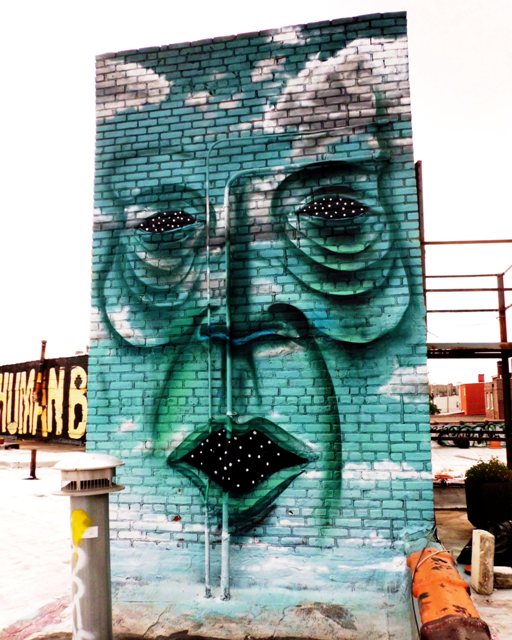In the center of an outdoor, potentially industrial area, stands a tall, narrow brick wall, reaching approximately 10 to 22 feet in height. The wall, which hints at a surrounding structure possibly hidden behind an elevated platform to its right, is adorned with a striking mural. The mural depicts a large, almost transparent face, rendered in shades of blues and greens. Across the face, fragmented white clouds dot the forehead, blending seamlessly into the sky-like hues of the face. The eyes and mouth, in stark contrast, are painted as cosmic black voids filled with scattering white dots, reminiscent of a star field or outer space. Below the eyes, sagging folds of painted skin droop towards a darker green nose and an open mouth mirroring the space theme. The surrounding environment, with visible graffiti and concrete elements, suggests a rundown, lower-income area, adding to the art's raw, gritty backdrop. To the left of the wall, a partially visible billboard or handmade sign reads "human" followed by a cut-off "B," and some scaffolding adds to the impression of an abandoned, urban landscape.